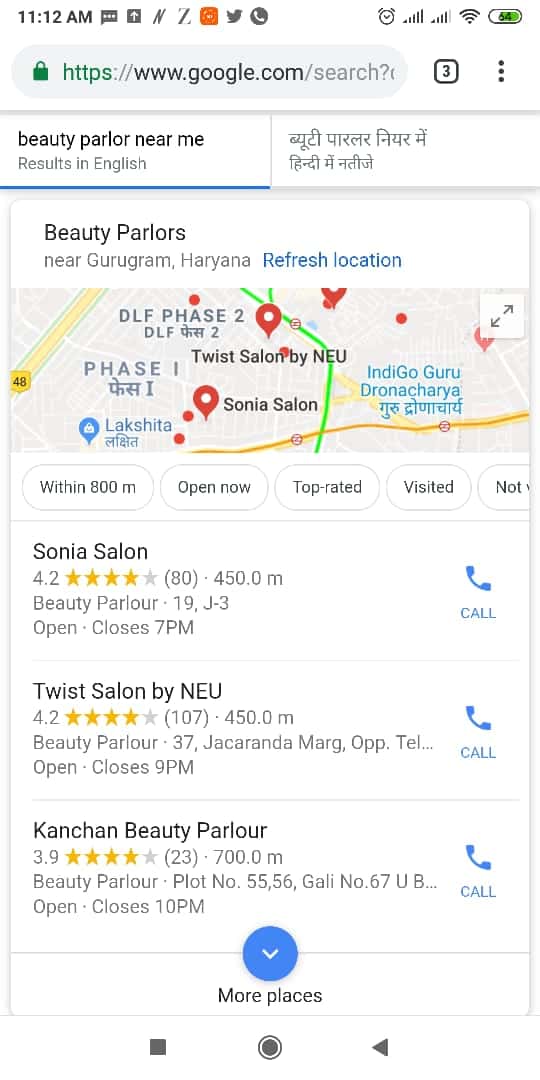This screenshot displays a Google search results page for "beauty parlor near me" with the user interface set to English. In the top left corner, the query is neatly presented. The screen features two tabs, with the second tab containing text in either Arabic or Sanskrit. Just underneath, a location update states, "Beauty parlors near Guru Gram, Haryana" next to a blue "refresh location" link. Dominating the central area is a map pinpointing the locations of "Twist Salon by NU" and "Sonia Salon" with bold red markers indicating their positions.

Further down, there are five pill-shaped filter buttons that allow users to refine their search by distance (within 800m), current operational status (open now), rating (top rated), personal visitation history (visited), and businesses not yet visited (not). Following this, three detailed business listings are displayed, providing information on each beauty parlor's name, rating, type, and closing time. Adjacent to each listing, users can find a blue call button for direct contact.